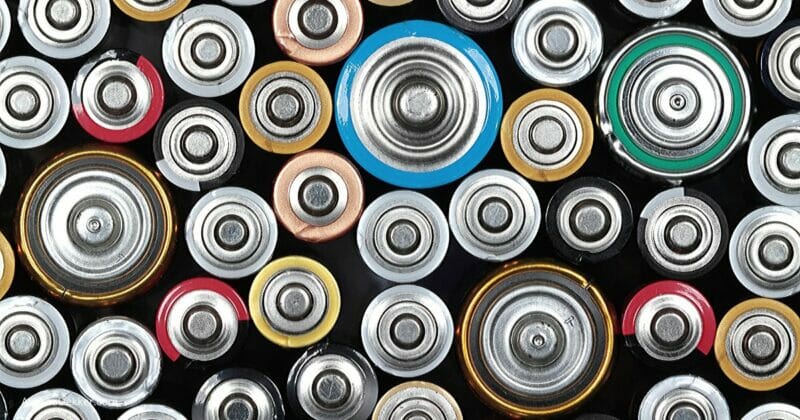This is a detailed image featuring a black background filled with variously sized batteries standing upright, showcasing their positive ends. The portrait-style photo captures the tops of these batteries, presenting a collage of colors and materials that resemble the cylindrical shapes of AA, AAA, C, and possibly D batteries. Each battery top displays a metallic, silver terminal encircled by different colored wrappings, including shades of green, light blue, red, silver, yellow, bronze, brown, and black. Some batteries bear similarities to Rayovac brands but lack any distinguishing text. The arrangement lacks a specific pattern, lending a random yet orderly appearance, with the tops outlined in black and highlighted by slight variations of white, light brown, and copper tones amidst the dark backdrop.